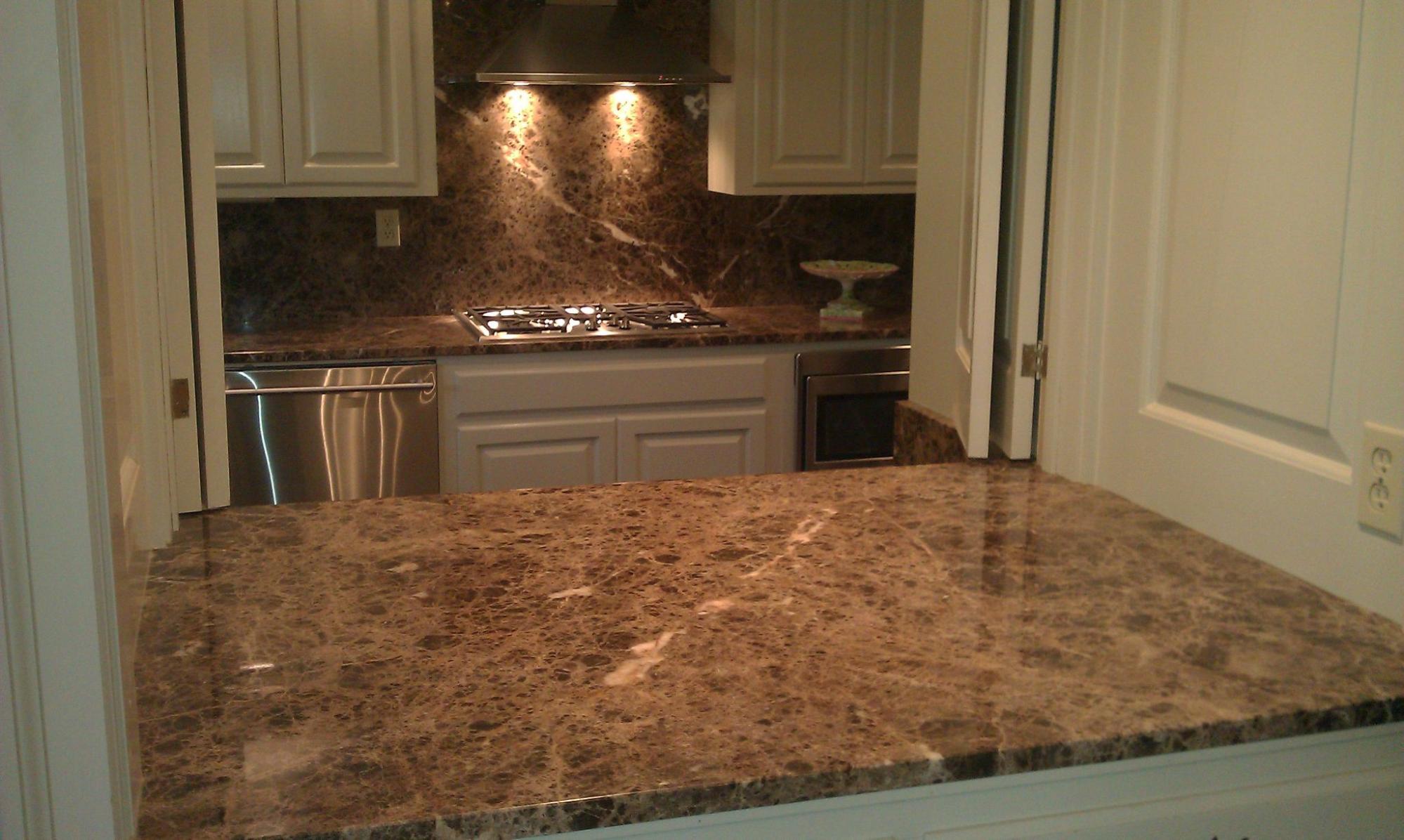The image captures a well-lit kitchen viewed from behind a brown and white marble countertop that serves as the foreground. In the background, the kitchen features an array of light tan or peach cabinets and shutters. Prominently, there is a stove top beneath an exhaust fan with overhead lights, casting a glow on the stainless steel appliances—the dishwasher to the left and a silver oven peeking from the right. Between these, a candy tray rests on the marble countertop. Above the stove, white cabinets provide storage, complemented by the consistent marble theme that extends both as a backsplash and additional counter space. The scene is framed by marble surfaces and a layout that appears to separate the kitchen from another room through white double doors, offering a detailed glimpse into a modern and stylish kitchen space.